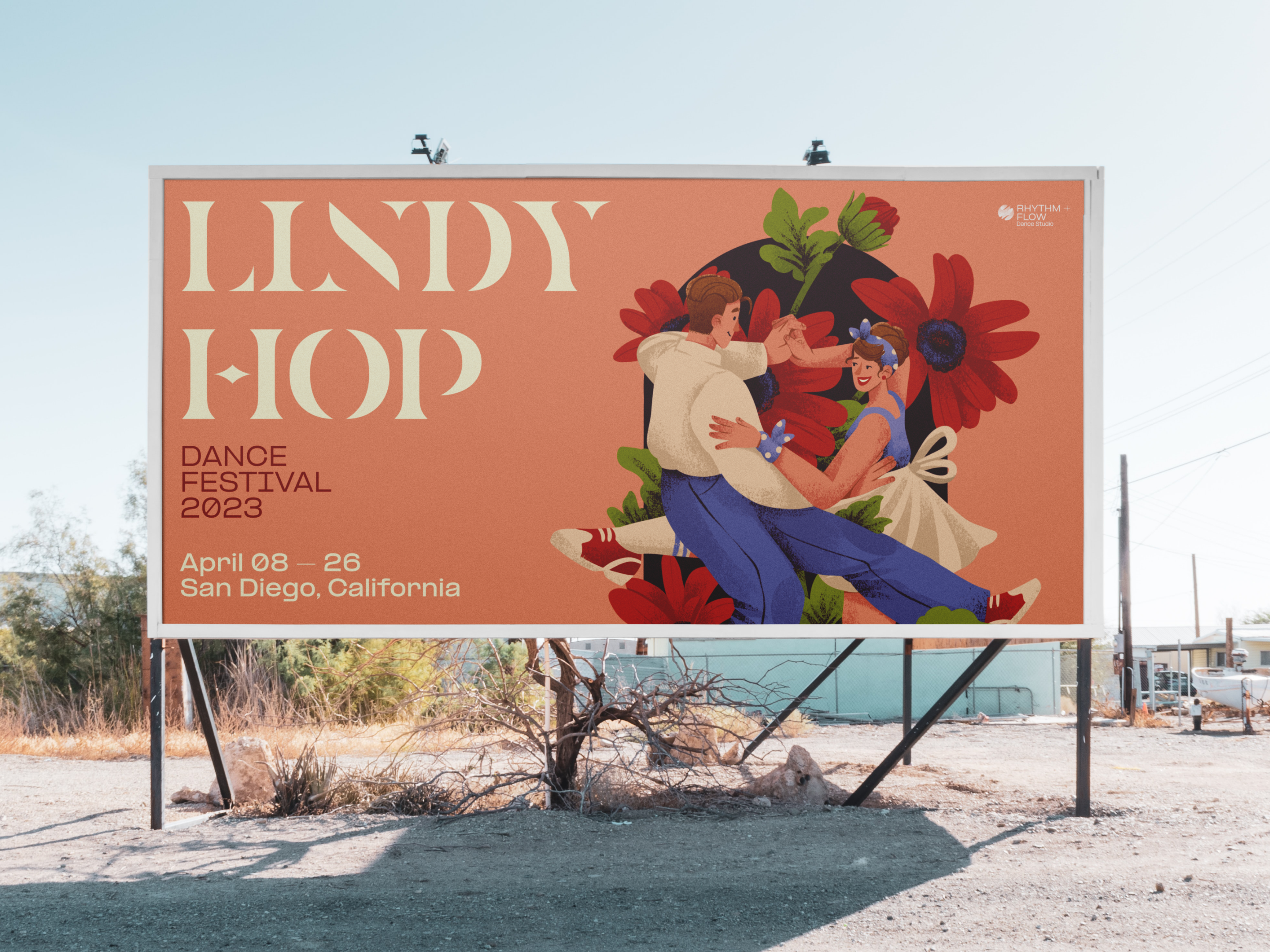The image features a large billboard set against a rustic, and somewhat desolate, landscape, revealed to be in a parking lot with hints of industrial buildings in the background. The expansive billboard stands tall with its posts firmly planted in the sandy ground. Dominating the sign are the words "Lindy Hop" in beige, set against a muted pinkish-orange backdrop. Below, in off-white and red lettering, the billboard announces the "Dance Festival 2023," which took place from April 8th to the 26th in San Diego, California. The billboard is vivid with a colorful illustration of a man and woman joyfully dancing. The man, dressed in blue slacks and a white dress shirt, and the woman, in a white skirt and blue tank top, both sport red sneakers. Surrounding the dancing couple, flowers in a black vase, specifically red carnations and green leaves, add a splash of charm. The scene is completed with additional, albeit unclear, white text in the top right corner. The composition suggests a celebration of energy, movement, and vibrant culture amidst the quiet and starkness of its surroundings.